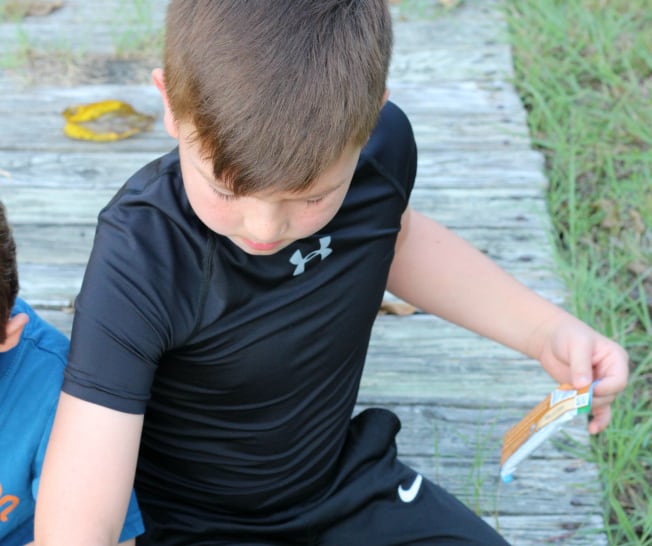A young Caucasian boy with light brown hair is sitting on a weathered grey wooden walkway with wood fibers running horizontally. Behind him lies a yellow leaf that is beginning to decompose, showing signs of brown. He is dressed in a black Under Armour t-shirt featuring a blue logo on the front, paired with Nike shorts that display a white swoosh. To his left stands someone in a blue t-shirt with black hair. The boy is holding a brown card with some numbers on it. On his right side, there is an area of tall green grass interspersed with a few leaves. Additionally, tufts of grass are growing between the wooden boards close to his left ear, adding a touch of nature to the scene.